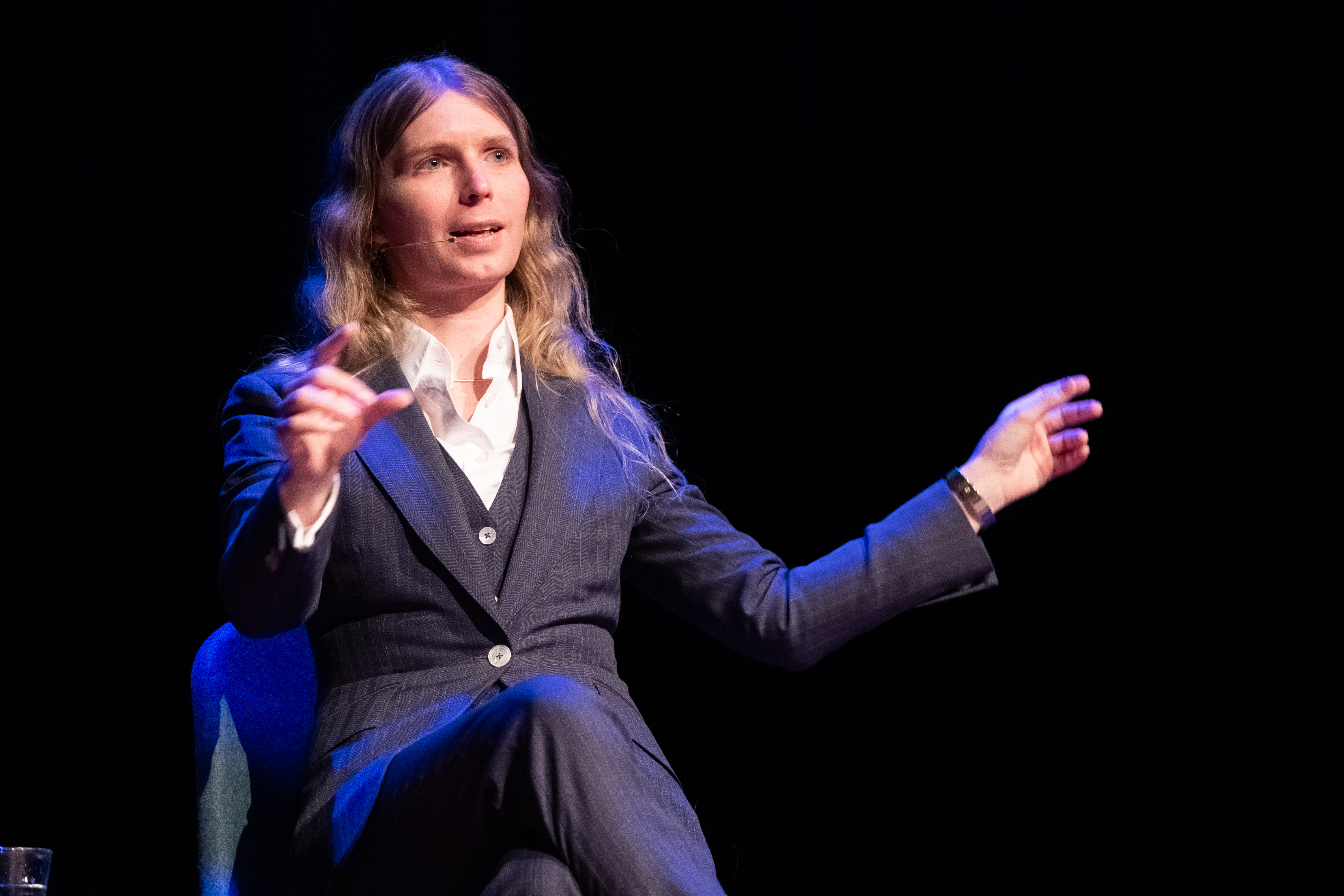The image features a young person with long, slightly wavy blonde hair parted in the middle, presenting in a professional setting. They are dressed in a pinstripe navy blue suit, complemented by a grey vest and white shirt. Sitting with their legs crossed on a darker-colored padded chair, they are making hand gestures while speaking to an audience, indicated by the small microphone attached from their ear to their mouth. The individual has an androgynous appearance, blending both masculine and feminine traits. A small glass of water is positioned to their lower left, and the scene is illuminated with a blue light shining from one side against a black background, giving the setting a TED Talk-like ambiance.